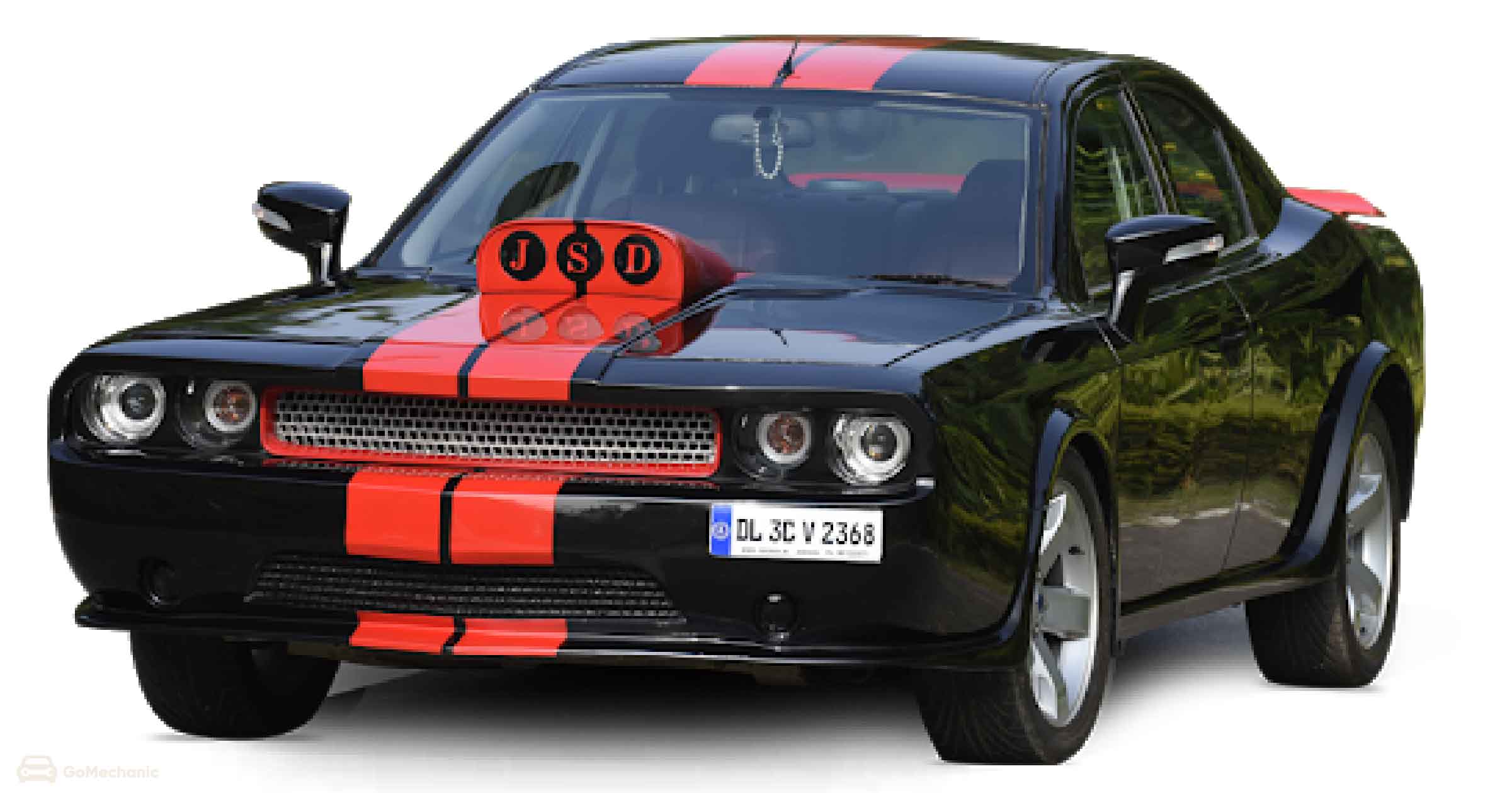This landscape-oriented color photograph features a sleek, black car with striking red racing stripes running down the center of the hood, across the top, and continuing to the rear, where a red spoiler is visible. The car exudes a nostalgic charm with its low-slung hood and broad, reflective surfaces capturing light reflections. It boasts a set of four round headlights, evenly distributed on either side of a wide, rectangular chrome grille outlined in red. The grille adds to the car's distinctive, somewhat aggressive front fascia. Positioned on the right side of the front bumper, the white license plate reads "DL 3C V 2368," accompanied by a vertical blue bar with a circle on it. 

A prominent feature on the hood is a raised scoop housing three black circles with red letters inside—J, S, and D. The dark interior is visible through the tinted windows, and a white necklace-like object dangles from the rearview mirror, though its details are obscured. Though reminiscent of a Dodge Challenger, the car has unique elements that suggest it might be a custom design. The background is stark white, creating a floating effect that highlights the car and accentuates its reflective surfaces, making it a centerpiece of photographic realism.